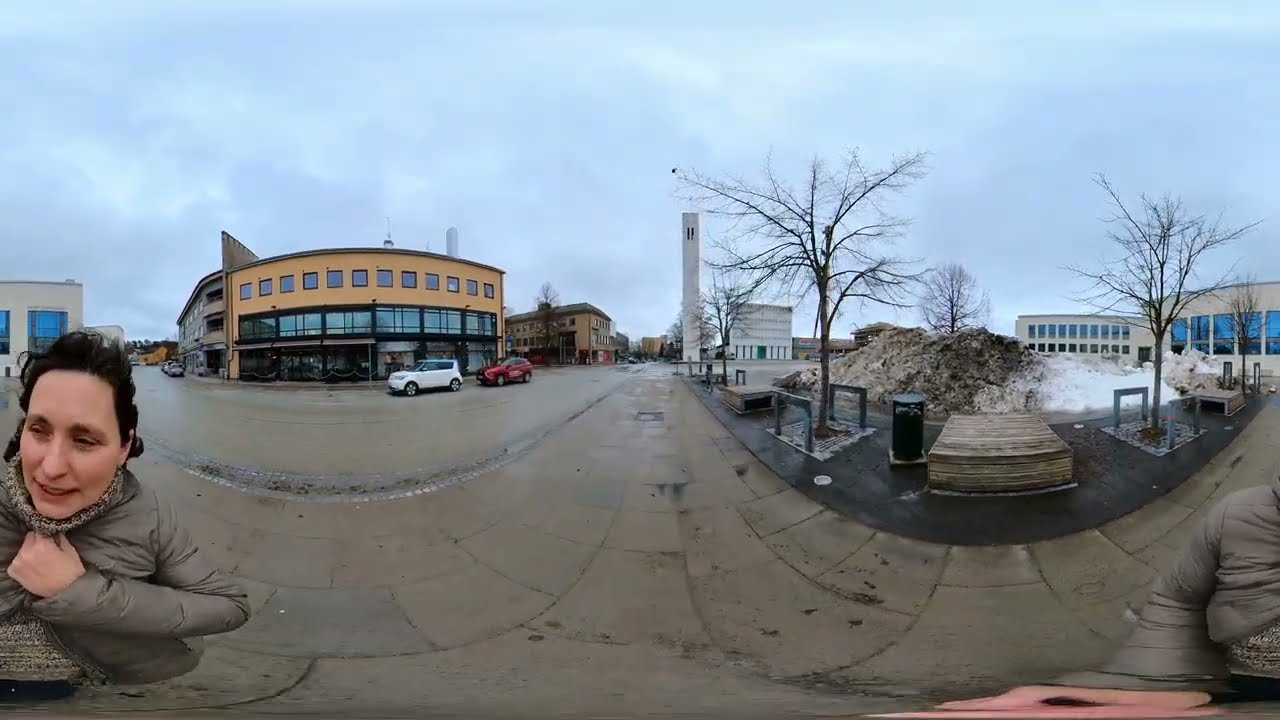In this 360-degree panoramic image, a woman in her 30s stands on a cement sidewalk next to a gritty pile of partially melted, plowed snow, indicative of a cold winter's day. Clad in a grayish-brown jacket and scarf, she clutches her scarf close to her neck with her left hand, suggesting she feels the chill, while her brunette hair blows in the wind. With her right hand, she holds a selfie stick attached to a 360-degree camera, looking slightly away from the viewer.

Behind her, the urban scene features a three-story building with a storefront on the bottom two-thirds, characterized by glass and black metal, and a brick top third. A couple of cars, including a white and a red one, are parked along the street. The right side of the image reveals a glimpse of a park with bare trees, benches, and a white tower, all under a cloudy sky.

The buildings in the background, appearing older with an industrial-chic aesthetic, suggest an area that has been gentrified with modern establishments like coffee shops or restaurants. The entire scene conveys a sense of a university area or a less busy part of town that has contemporary charm amidst the starkness of winter.